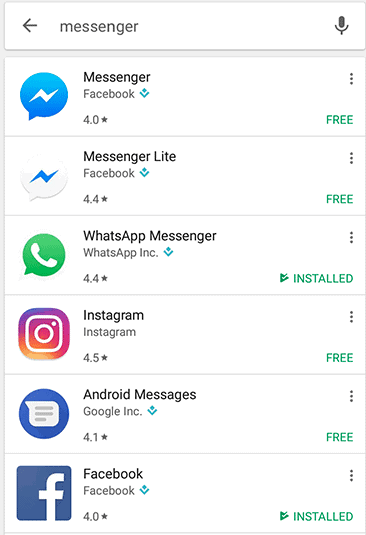**Screenshot of Mobile App Search Results:**

The screenshot displays a search result page within a mobile app store, characterized by a light gray background. At the top of the screen, an input bar is prominently featured. Inside this input bar, the word "messenger" is entered. To the right of the input bar is a dark gray microphone icon, while to the left is a gray back button.

Below the input bar, six white rectangular bars are listed vertically, each representing a different app associated with the search query. Each rectangle contains the app's name, rating, installation status, and logo:

1. **Messenger for Facebook**: Rated 4.0 stars. The app is free (indicated by green text), and its logo is blue with a white lightning bolt.
2. **Messenger Lite (Facebook)**: Rated 4.4 stars. This app is also free, with a logo similar to Messenger but with inverted colors.
3. **WhatsApp Messenger**: Rated 4.4 stars and shown as installed. The logo is a green speech bubble with a white phone icon.
4. **Instagram**: Rated 4.5 stars. This app is free, featuring the Instagram logo with a camera icon.
5. **Android Messages (Google Inc.)**: Rated 4.1 stars. This app is free, displaying a blue text message bubble logo.
6. **Facebook**: Rated 4.0 stars and marked as installed.

The highlighted details provide a clear understanding of each app's popularity, availability, and visual identity.